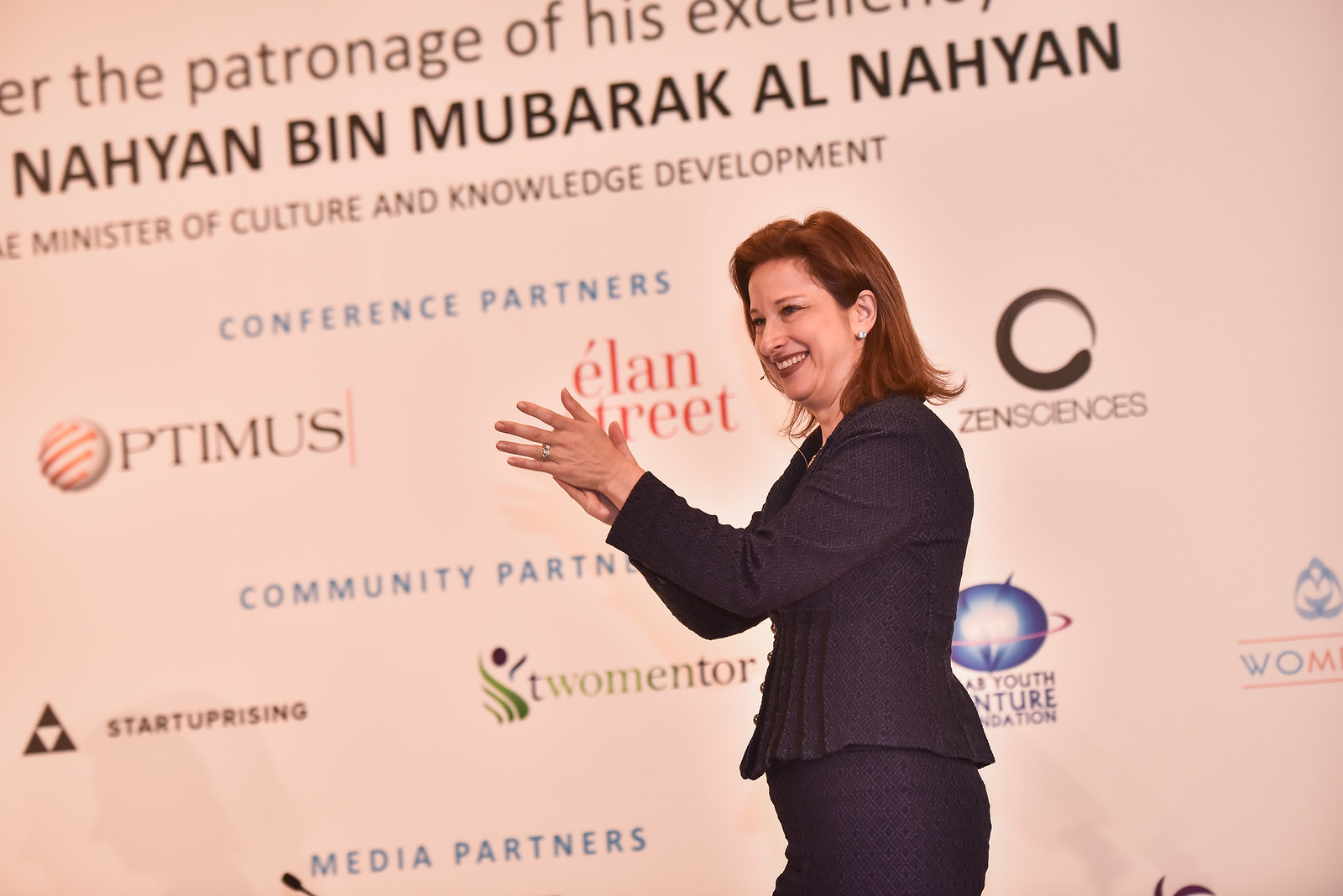The full-color photograph captures a middle-aged woman standing on a stage indoors at a professional event. She is smiling broadly and appears to be clapping, suggesting she might be acknowledging or presenting an award. The woman has shoulder-length brown hair and is dressed in a classic blue business suit consisting of a jacket and a skirt. The backdrop behind her features partial text that reads, "The patronage of his excellency, Nayan bin Mubarak Al Nahyan, Minister of Culture and Knowledge Development," alongside a list of conference sponsors and media partners. Some of the visible sponsor names include Optimus, Elan Street, Zen Sciences, and Start Uprising, though several names are obscured. The image is clear and well-lit, with no other individuals or objects in the frame, emphasizing the woman's prominent and enthusiastic presence on stage.